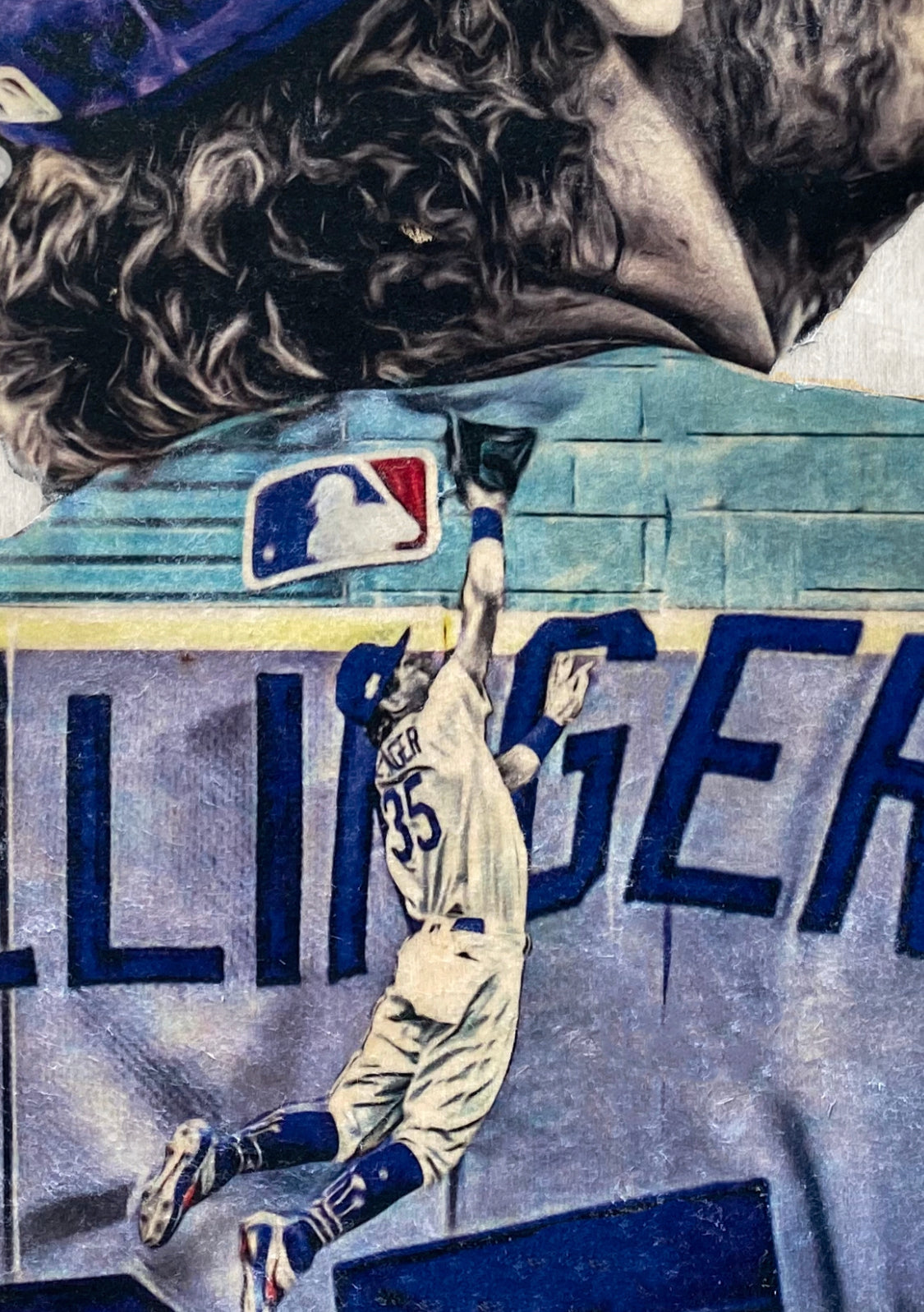The illustration depicts a baseball player in a dynamic pose, reaching high with his right hand, glove in tow, attempting to catch a ball. Clad in a white and blue uniform, number 35, and a blue cap, the player is prominently featured in the bottom half of a vertical rectangular frame. He stands out against a backdrop comprising a blue cinder block wall adorned with a blue and white cloth banner. Above the irregular edge of the wall, there is a stylized depiction resembling a bird's beak enveloped in curly feathers. A rectangular object with rounded corners, displaying a white silhouette of a baseball player, is also affixed to the wall. The mural-like quality of the artwork is underscored by a mix of painting and slight animation effects, creating a vivid, almost lifelike scene. Large letters, part of the background, spell out fragments of a name, possibly "L-I-N-G-E-R," suggesting another player's name or team branding. The fence near the bottom transitions from a purplish hue to a light blue brick pattern, adding layers of depth and color to the scene.